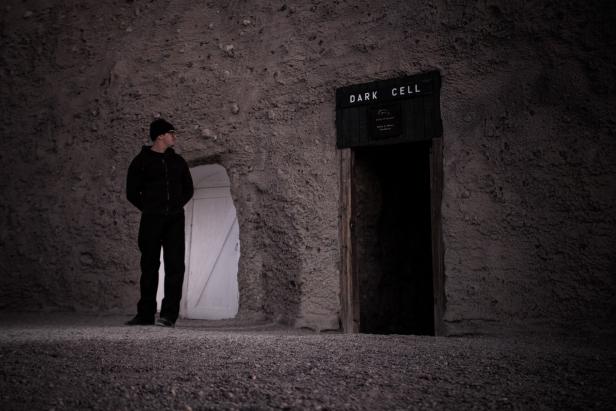The photograph depicts an underground scene, resembling the interior of a cave or mine, with a rocky, carved-out background. The ground is covered in dirt, and prominent structures emerge from the rock formation. On the left side, a man dressed entirely in black—including a hoodie, pants, shoes, and a beanie—stands with his body facing forward but his head turned to the right. His hands are in his pockets, and he appears to be contemplating. The left section of the image reveals a small doorway carved into the rock, displaying a white interior. To the right, there is another carved opening supported by wooden beams, with a black rectangle above it that reads "DARK CELL" in white text. This doorway leads into pitch darkness. The contrasting elements and the man's pensive posture contribute to a sense of curiosity and contemplation within this somber, subterranean setting.